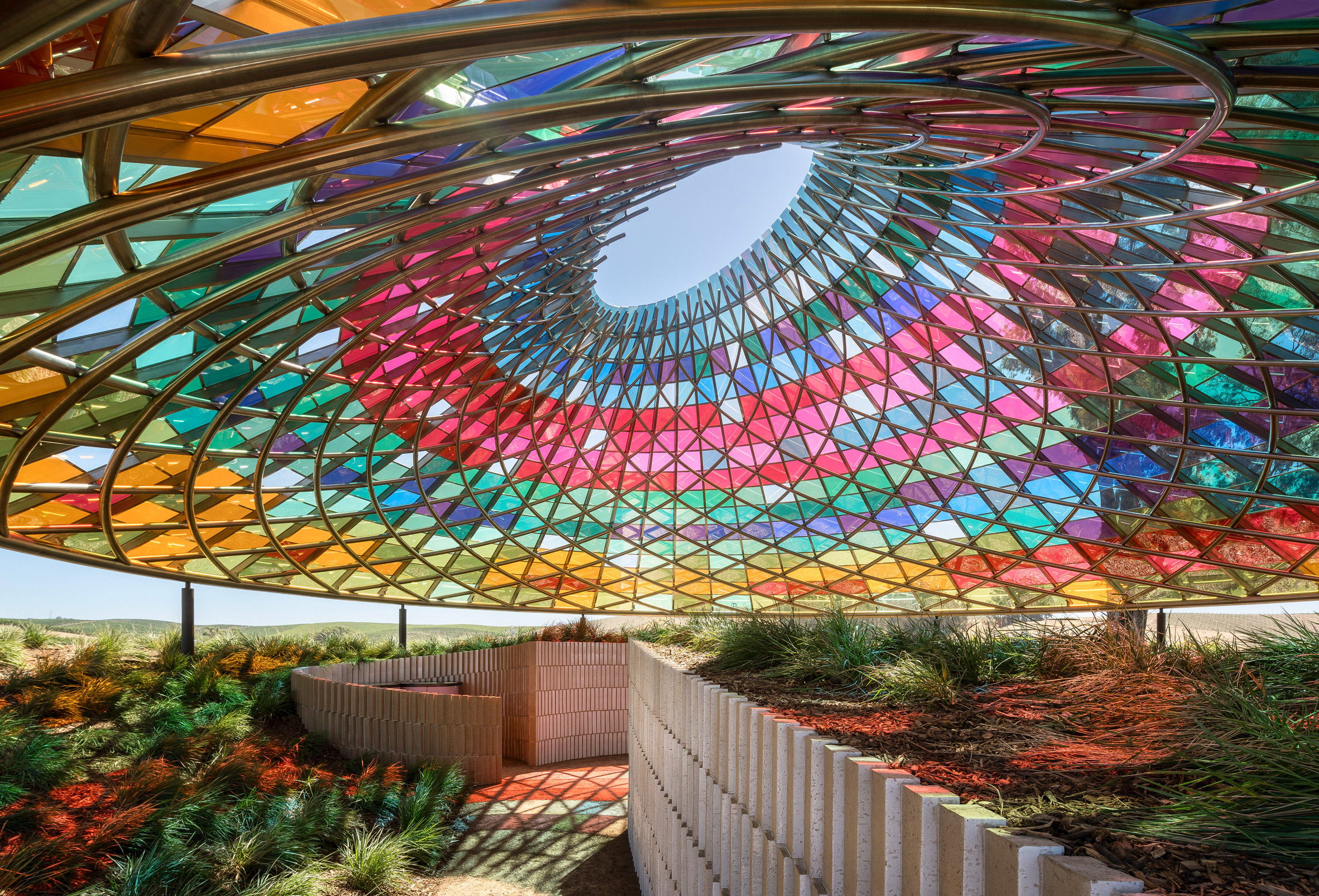The image depicts a striking computer-generated scene featuring a vast, dome-like structure seemingly set in an open field with rolling hills and an expansive blue sky in the background. A magnificent glass and metal lattice roof dominates the frame, curving gracefully with an intricate grid pattern. The metal framework, with its shiny copper hue, twirls upward to form a circular, concave roof with an oval-shaped opening at the apex, allowing a glimpse of the sky above. The roof comprises a spectrum of stained glass panels, displaying a dazzling array of colors that transition from warm yellows and oranges at the base, through reds and pinks in the middle, to purples, greens, and light blues towards the top.

Beneath this vibrant canopy, the scene includes neatly maintained walkways bordered by stone brick walls and retaining structures. These walls feature raised garden beds, where diverse plant species thrive, adding a touch of greenery to the metallic and glass surroundings. The pillars supporting the roof enhance the open-air design, ensuring an unobstructed view of the serene plains spreading out beyond the structure. The sunlight filtering through the multi-colored glass projects a beautiful, kaleidoscopic silhouette of colors onto the ground beneath, creating an enchanting and visually captivating atmosphere.